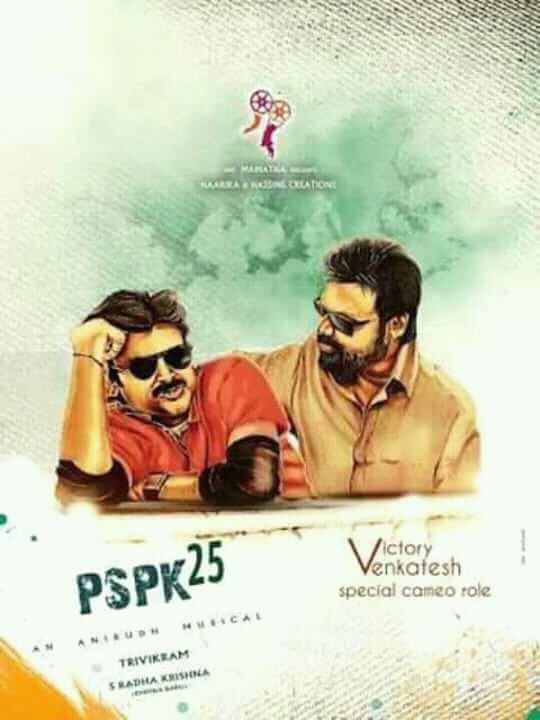The image is a poster for a musical titled "Anabush," primarily featuring two men seated in the center. The poster has a stylized, illustrated appearance rather than a photographic one. The background consists of predominantly greenish and bluish hues with cloud-like visuals dominating the upper portion. 

The man on the left is engaged in conversation, with mid-sentence expression, and is dressed in a red short-sleeved shirt adorned with black elbow pads. He wears a watch on one wrist and a band on the other, complemented by black sunglasses and sporting dark brown hair with a matching mustache. His head is supported by his hand, resting on his elbow.

The man on the right is more passively watching his companion, attired in a yellowish-beige button-down collared shirt, and like his counterpart, he wears sunglasses. He has dark hair and a full beard.

Occupying the lower part of the poster, significant text includes "PSPK 25" where the number "25" is slightly raised, indicating a notable milestone. The prominently large "V" followed by the smaller text "Victory Venkatesh" hints at a special cameo role by the individual. Further confirmation of this is provided by the phrase "special cameo role" in smaller text.